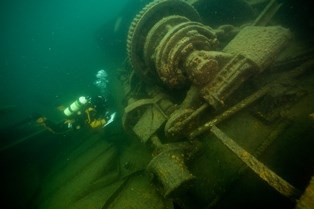The image captures an underwater scene where a scuba diver, dressed in a black wetsuit with red accents and equipped with a white and yellow air tank, is inspecting a large metallic machine encrusted with corrosion. The diver, positioned slightly left of center, is emitting bubbles from their face mask as they use an equipment with a light to examine the object. The primary focus is a large gear, wider than the diver is long, which suggests the remains of a rotational engine apparatus, likely part of a sunken shipwreck's generator or turbine system. Surrounding this machinery are various mechanical components, adding to the intricate details. The atmosphere of the photograph is dark and murky, indicating the scene is at a considerable depth, and achieving a high level of detail is challenging due to the dim natural light and the underwater conditions.